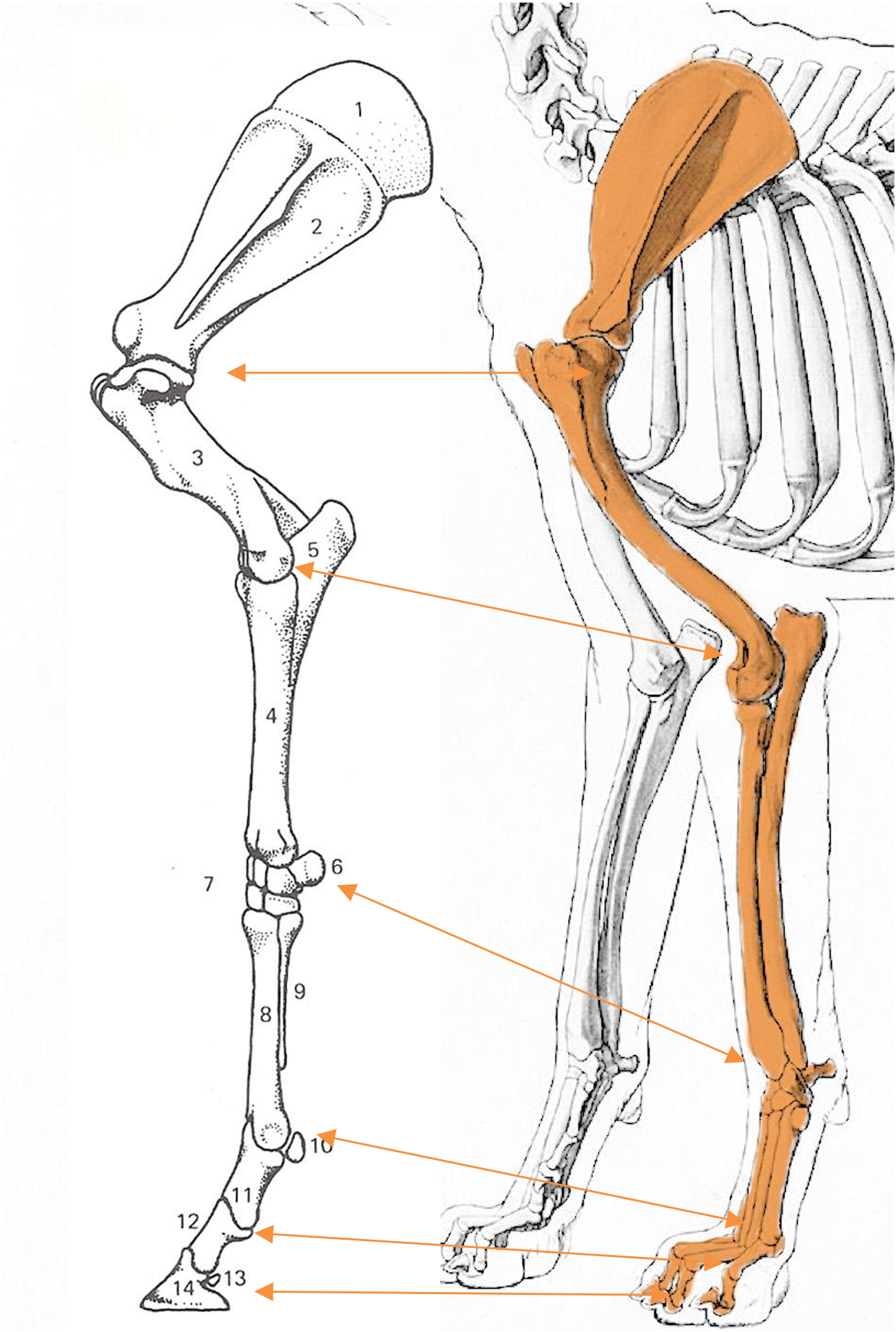This is a detailed scientific diagram depicting the skeletal structure of a horse, specifically focusing on the leg bones. The illustration, rendered in black and white line art, includes the rib cage, hip bones, and neck outline. On the right side, the diagram offers a simplified skeletal outline of the horse, with one leg highlighted in a distinctive light orange color. On the left side, this highlighted leg is drawn in greater detail, showing individual bones meticulously labeled and numbered from 1 to 14 from the top down. Thin orange arrows extend from the orange-colored leg on the right to their corresponding detailed parts on the left, illustrating the relationships between different bones in both the front and back legs of the horse.